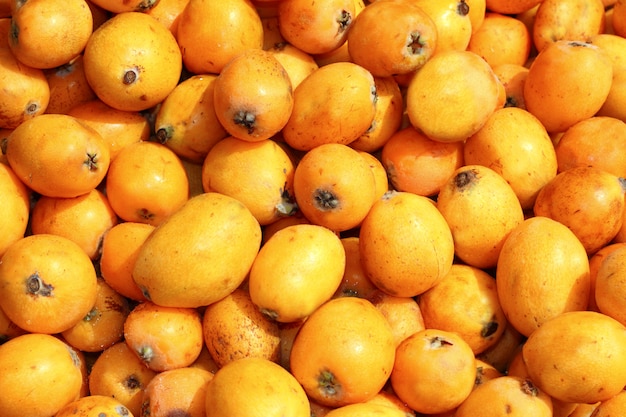The image features an abundance of fruit, likely loquats or possibly persimmons, piled generously as they would be in a bin or on a produce aisle. The fruits are predominantly yellow with brown ends, and they exhibit a spectrum of yellowish-orange hues. Each fruit, about one to two inches in length, varies in shape from round to oval, and some even appear to have a bell shape. They possess a luminous, tough skin that shines brightly in the well-lit photo, making them look ripe and very appetizing. Many of the fruits display stem ends, while a few bear minor bruises or brown marks. The fruits seem freshly picked, with an unwashed, natural appearance, enhancing their visual appeal in this high-resolution, vibrant snapshot. This detailed and appealing scene could easily be mistaken for a green grocer's abundant and fresh offerings.